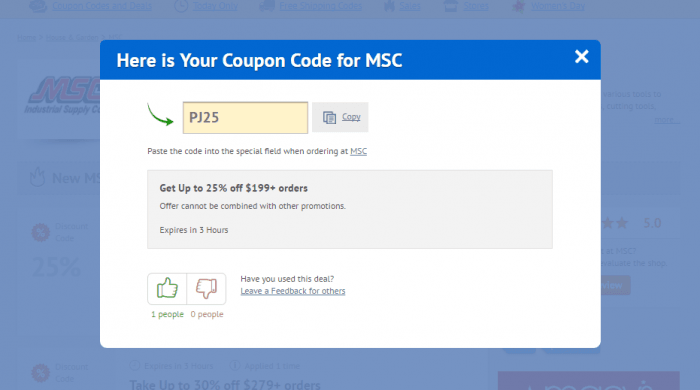On this page, you will find important text regarding a special promotion. Here is your exclusive coupon code for MSC: PG825. To utilize this offer, simply paste the code into the designated field when placing your order on the MSC website. This coupon grants you up to 25% off on orders of $199 or more. Please note that this offer cannot be combined with other promotions and expires in 3 hours. We encourage you to share your experience if you have used this deal, as your feedback could be valuable to others. There are additional details regarding this promotion in the image, though they are not fully legible.